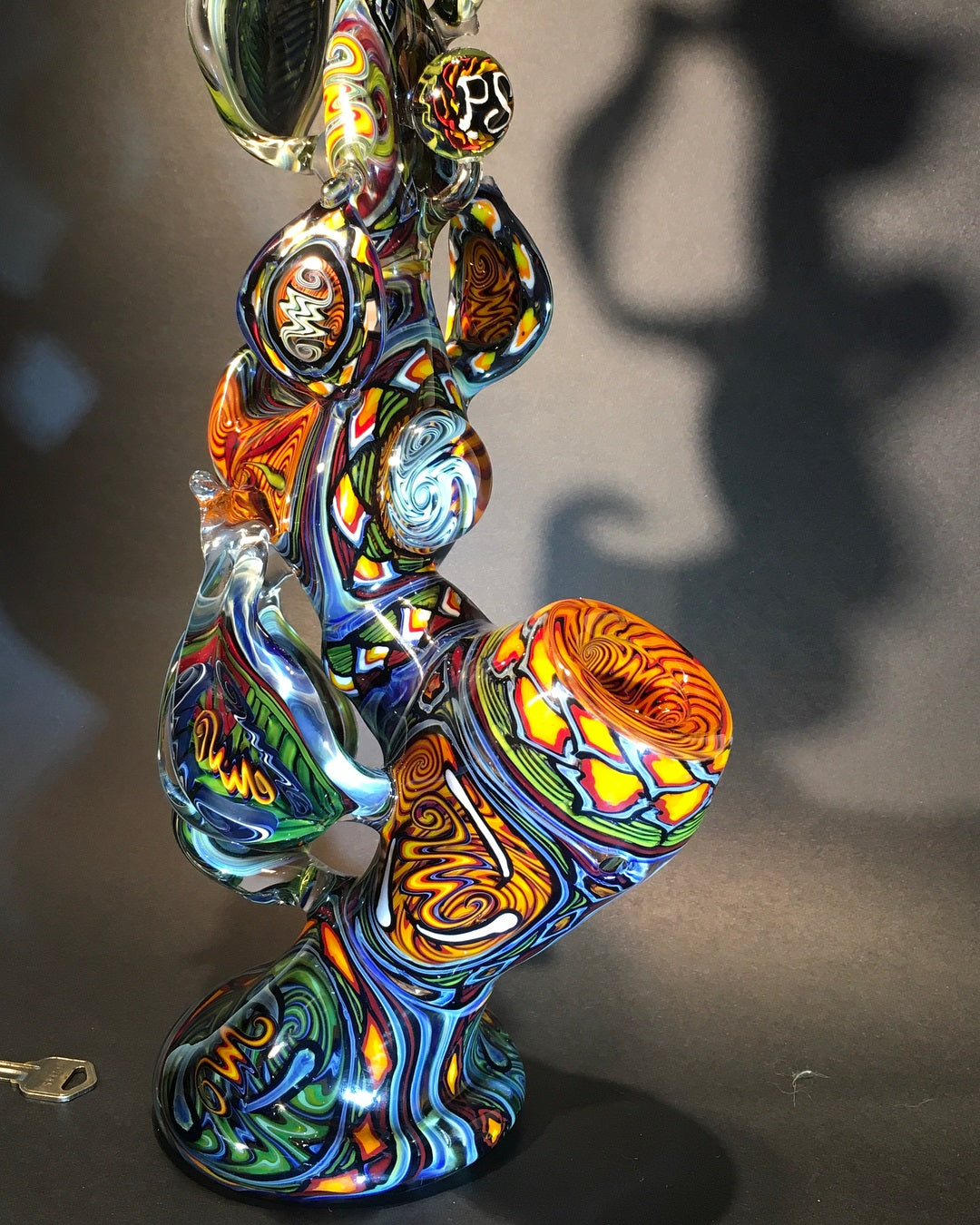The photograph showcases an intricate piece of glass artwork positioned on a dark gray surface that seamlessly extends up the wall behind it. In the bottom right corner of the surface, small white fuzz is noticeable, adding a subtle detail to the scene. To the bottom left, a silver house key lies adjacent to the glass artwork, possibly to provide a sense of scale. The tall, ornate glass piece features a flared base and is adorned with a mesmerizing swirl of green, blue, orange, and white colors. Its knobby structure includes sections resembling leaves that branch out from the main form. The top of the artwork extends beyond the frame, leaving it partially visible. Illuminated by light, the glass piece casts a distinct shadow on the wall, enhancing its intricate textures and vivid colors.